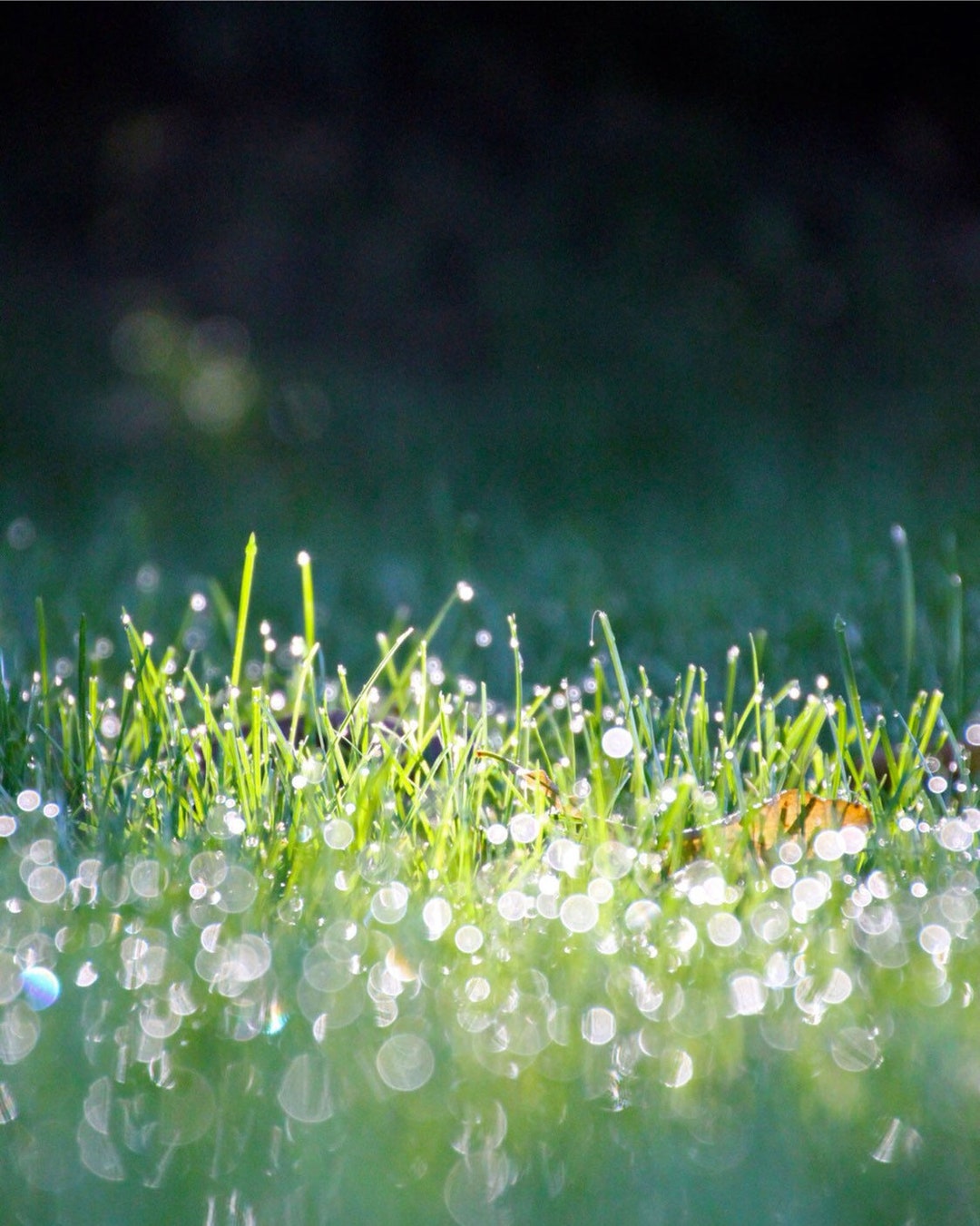A close-up photograph captures the delicate beauty of dew-covered grass at ground level. The focal point of the image reveals sharp, green blades of grass adorned with glistening dew droplets, which resemble small, white, reflective spheres. The foreground and background of the photo are blurred, creating a striking contrast that highlights the central blades of grass. These droplets, illuminated by abundant sunlight, create a shimmering effect. Scattered among the grass is a lone, reddish-orange leaf, adding a pop of color to the verdant scene. The backdrop features softly muted, dark green trees, enhancing the ethereal quality of the photograph. The overall composition evokes a feeling of early spring, with new grass emerging and the sun casting a gentle glow on the morning dew.